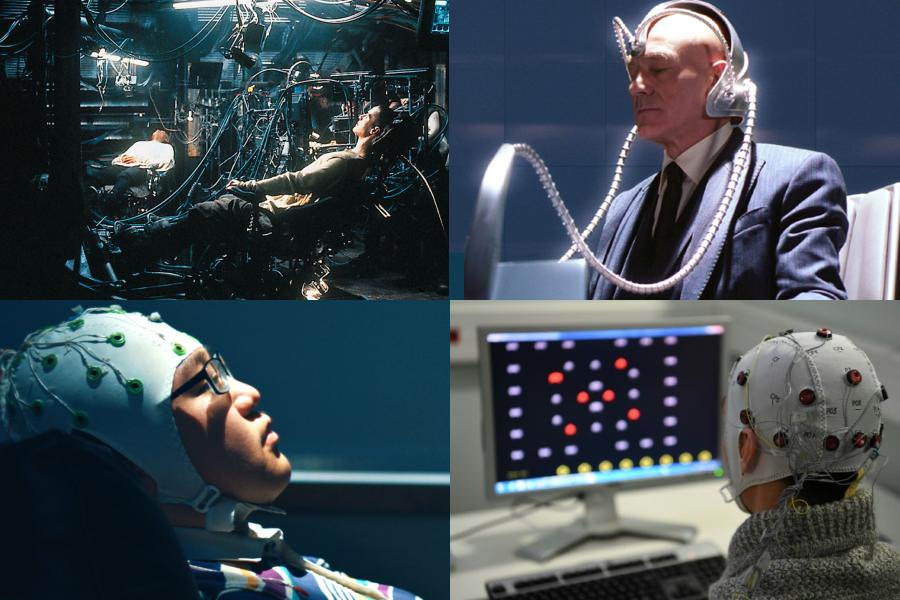This color photograph is neatly divided into four sections, each portraying a different aspect of what appears to be a scientific study. 

**Top Left**: The first segment is a dimly lit room where two men are lying down in fully reclined chairs that resemble beds. Both individuals are connected to numerous wires and hoses. One man is dressed in a white shirt, while the other wears a tan shirt. The room's darkness and the abundance of wires create a scene reminiscent of a science fiction movie.

**Top Right**: This section features a well-dressed gentleman in a three-piece suit and tie. He has a silver metallic device on his head that encircles his forehead and ears. This device includes two elongated, snake-like wires that extend towards a point in front of him.

**Bottom Left**: Here, an Asian man with glasses is depicted wearing a rubber cap fitted with electrodes or similar connectors. The significance of this setup suggests it could be related to brainwave monitoring or some type of neuroimaging.

**Bottom Right**: The final segment shows another individual with a similar electrode cap, positioned in front of a computer monitor displaying various colored dots. This person appears to be engaged in a task or test, indicative of a controlled experimental setting.

Together, these images create a comprehensive view of a complex, technology-driven scientific experiment involving human subjects.